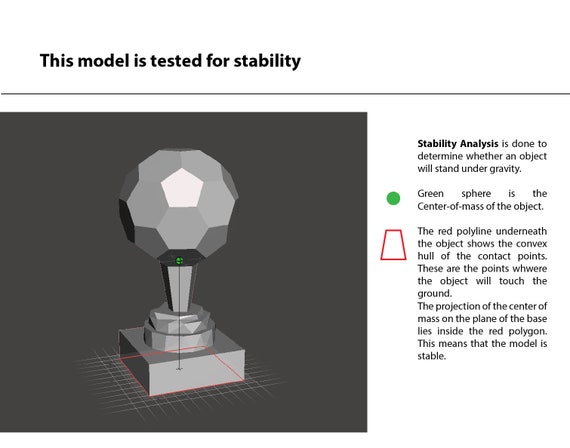The image is a detailed black and white schematic or diagram, likely sourced from a textbook or website, illustrating the stability analysis of a 3D geodesic sphere model, which resembles a metallic soccer ball with hexagonal facets. The model sits atop a tapering cylindrical structure that transitions to a craggy base, which then rests on a circular platform atop a larger square base, all positioned over a grid.

This diagram is labeled at the top with the text, "This model is tested for stability," and it explains that the stability analysis determines if an object can stand under the influence of gravity. Central to the analysis is a green dot representing the center of mass, located at the base of the geodesic sphere. Furthermore, a red polyline beneath the object illustrates the convex hull of the contact points, indicating where the object will touch the ground.

The projection of the center of mass onto the plane of the base falls within the red polygon, confirming that the model is stable. This comprehensive schematic visually demonstrates how the center of mass and the convex hull of contact points correlate in assessing the model's stability under gravitational forces.